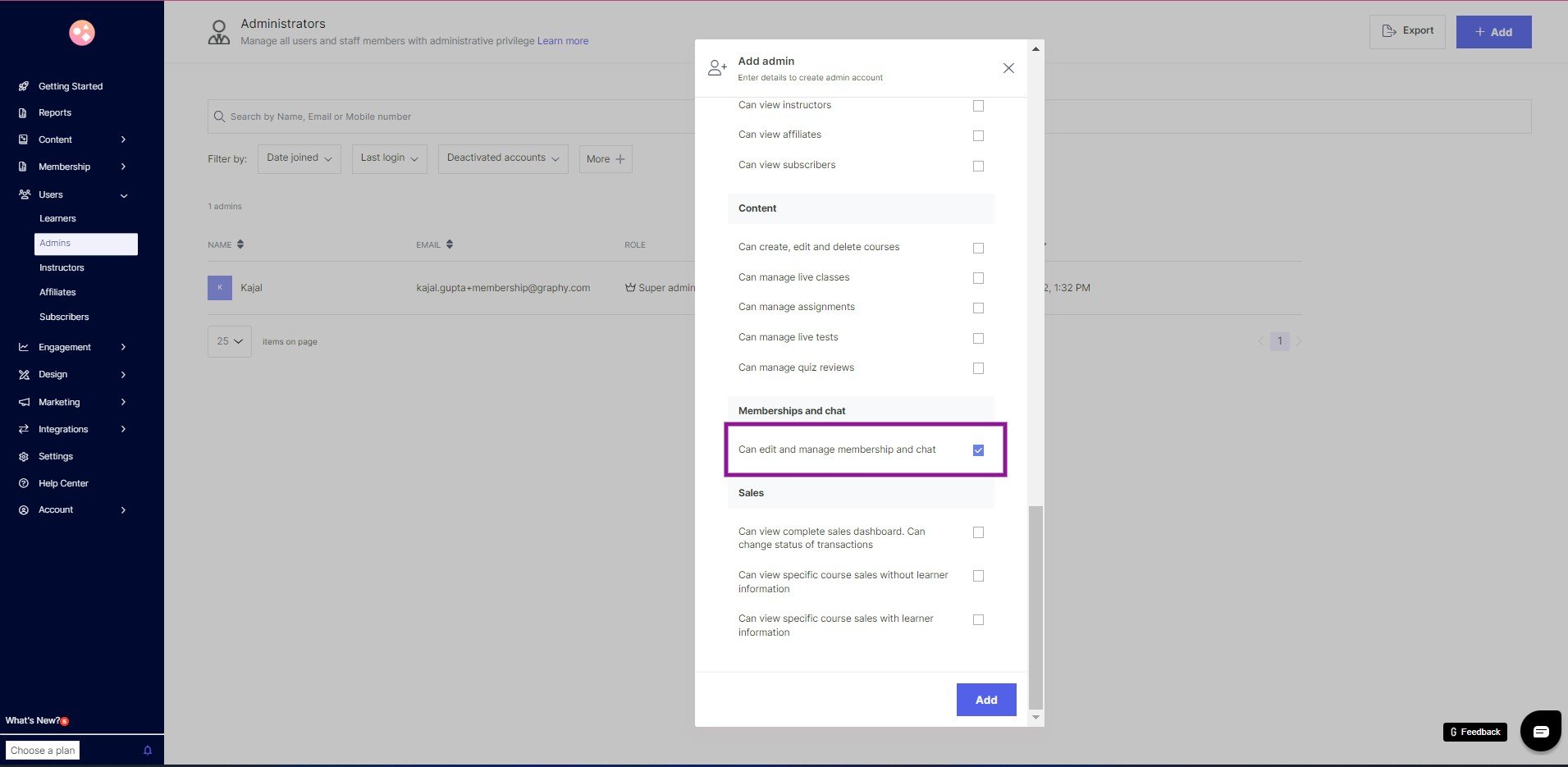This image captures a screenshot of a web page, presumably from a user management platform intended for administrators. At the top of the page, there is a section labeled 'Administrators,' accompanied by a description that reads "Manage all users and staff members with administrative privileges." Adjacent to this, highlighted in blue, is a "Learn More" link.

Running vertically along the far left side of the screen, there is a black sidebar filled with clickable icons and labels. At the very top of this sidebar, there is a circular icon containing a square, circle, and triangle with an adjacent rocket icon labeled "Getting Started." Below this, there are additional icons each paired with descriptive text, including a white paper labeled "Reports," a TV labeled "Content," and several more categories: Membership, Users, Learners, Admins, Instructors, Affiliates, Subscribers, Engagement, Design, Marketing, Integrations, Settings, Help Center, Account. Notably, at the very bottom, there is an entry labeled "What's New," marked with a red circle. Additionally, at the bottom left corner, a white box prompts users to "Choose a Plan."

The main content area of the page is predominantly gray, featuring several open boxes. One of these boxes is outlined in purple and encompasses text related to user permissions, stating, "can edit and manage membership and chat."